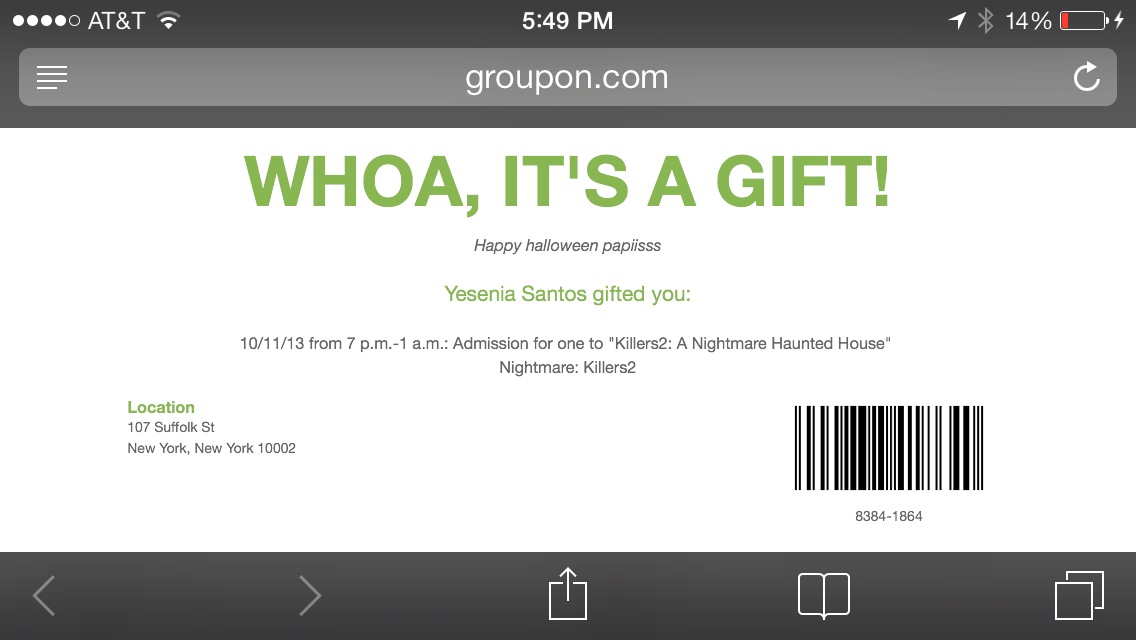This is a landscape-oriented screenshot of an iPhone showing a browser app open to Groupon.com. The carrier, AT&T, is displayed on the top left, with a Wi-Fi signal strength indicator showing two bars, and a battery level at 14% with a lightning symbol. The time is 5:49 p.m. The webpage features large green text at the top that reads, "Whoa, it's a gift. Happy Halloween, PAPLISS." Beneath this, in smaller green text, it says, "Yesenia Santos gifted you 10-11-13 from 7 p.m. to 1 a.m., admission for one to Killers 2, a nightmare haunted house, Nightmare Killers 2, location 107 Suffolk Street, New York, New York, 10002." There is also a barcode visible in the bottom right corner of the screen.